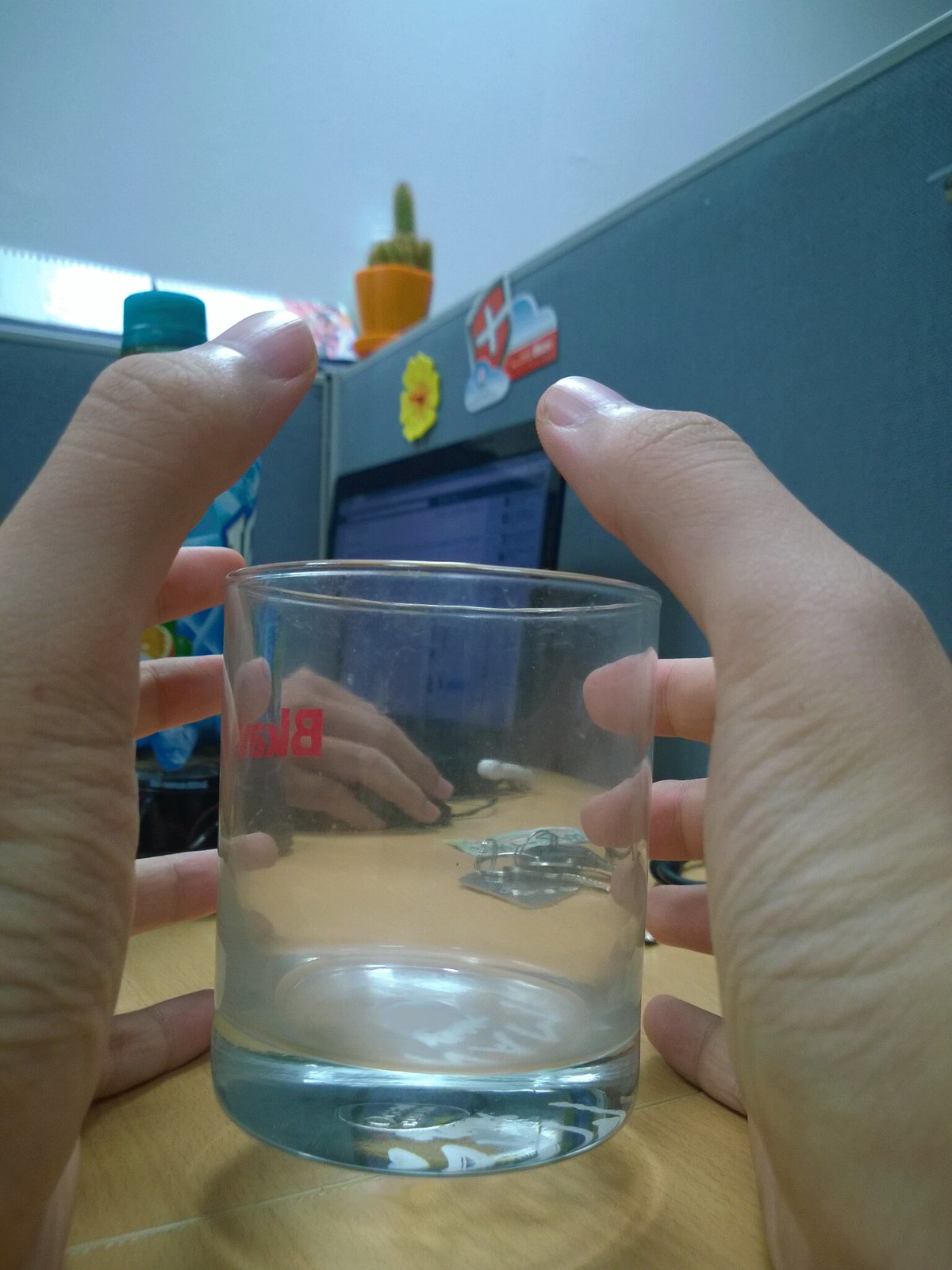In this detailed indoor office cubicle scene, a glass cup appears to be levitating about an inch above a brown wooden table, framed by a person's tensed hands with fingers outstretched but not touching the glass. The glass, which resembles a rocks glass and features an indistinguishable red logo with the letter 'B', has a shadow beneath it enhancing its floating illusion. The background reveals a black laptop screen, a hand on a mouse, and other cubicle elements including a cactus at the intersection of cubicle dividers, along with various stickers on the walls. The scene is captured in a rectangular photograph, emphasizing the mysterious hovering glass as the central focus amidst a typical office setting.